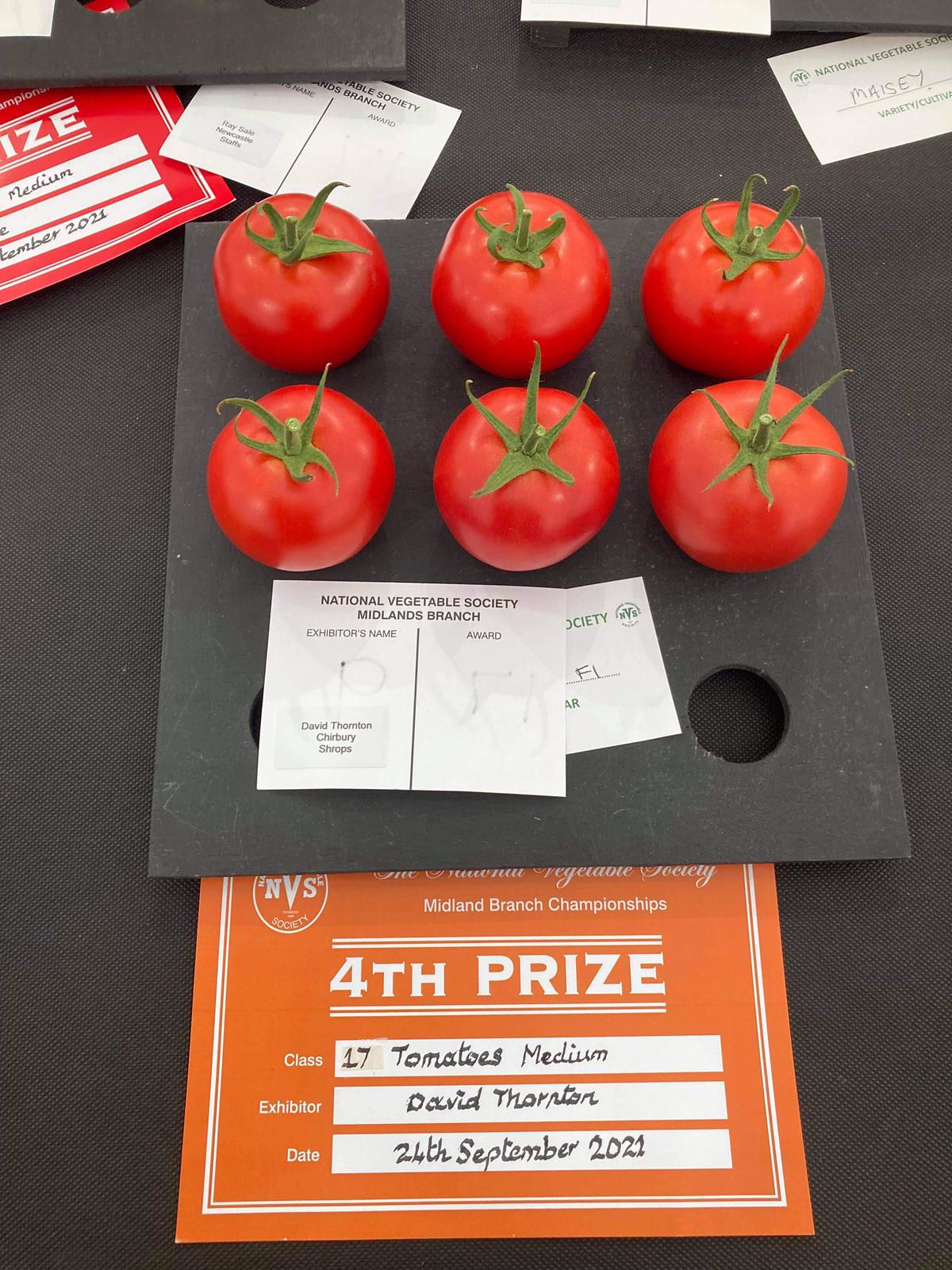The image showcases six vibrant, medium-sized tomatoes, each about the size of a woman's fist, elegantly arranged in a black tomato holder on a black table. These tomatoes, which took fourth place in the National Vegetable Society's Midland Branch Championship on September 24, 2021, were grown by David Thornton. His award is highlighted by a prominent orange certificate detailing his placement in Class 17 – Medium Tomatoes. Surrounding Thornton's impressive display are additional certificates and awards from other contestants, creating a backdrop that emphasizes the competitive nature of the event. The bright red tomatoes, with their decorative green tops, stand out as a testament to Thornton's horticultural skill, despite the notable presence of other prize-winning entries.